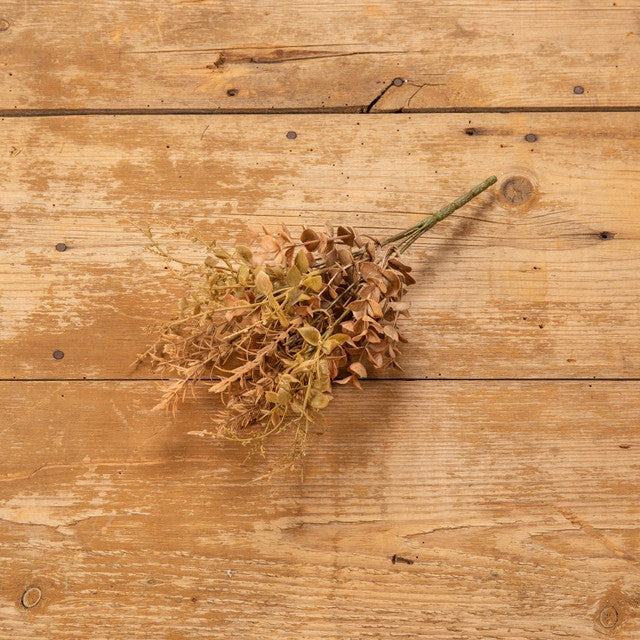In the image, a dried and decayed plant sits prominently on an aged, untreated wooden table with three uneven two-by-four planks, displaying visible cracks, knots, and scratches. The wooden surface, rich in texture and imperfections, serves as a complex backdrop to the plant, which features an olive-green stem and spiky brownish leaves that closely match the wood's color. Some leaves even verge towards a yellowish hue, enhancing the impression of desiccation. Positioned centrally on the table, the plant—with its long, skinny stems and numerous small leaves—creates an intriguing visual contrast between natural decay and synthetic mimicry, suggesting it is a piece of artificial foliage. There's no text present in the image, leaving the scene to speak entirely through its visual elements.